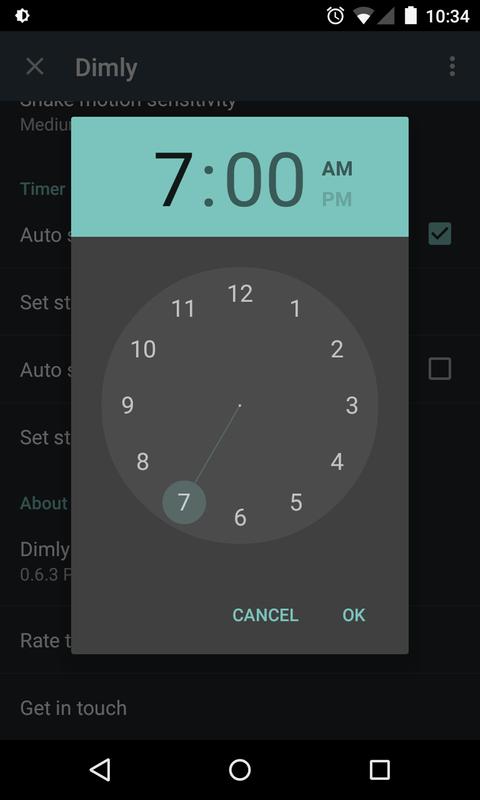The image is a screenshot taken of someone’s phone displaying the alarm settings screen. 

At the very top, there is a thin black status bar. On the right side of this bar, you can see several icons: a clock representing the current time, a signal icon for Wi-Fi connectivity, a triangular warning or signal strength indicator, a battery icon showing the battery level, and the time "10:34" in white text.

Below the status bar, there is a thicker dark gray header with a lighter gray "X" on the left side and the word "dimly" next to it, written in lowercase letters.

The main section of the screen is divided into two parts. The top part is light blue and prominently displays a large black number "7" followed by a colon and "00", both in gray. Above this time, in a darker gray, are the letters "AM". The letters "PM" are displayed in a much lighter gray color next to "AM".

The bottom part of the screen is a light gray color and features a circular clock face with numbers 1 through 12 displayed in white. A line extends from the center of the clock to the number "7," which is circled. Below the 6 on the clock, there are two buttons: "Cancel" in all capital letters and baby blue, and "OK."

In the background, partially visible, are other settings options such as "timer" and "auto-set", indicating that this screen is part of a larger settings menu where the user can adjust different time-related settings.

Overall, the image captures the detailed layout and design of the alarm settings interface on the user’s phone.